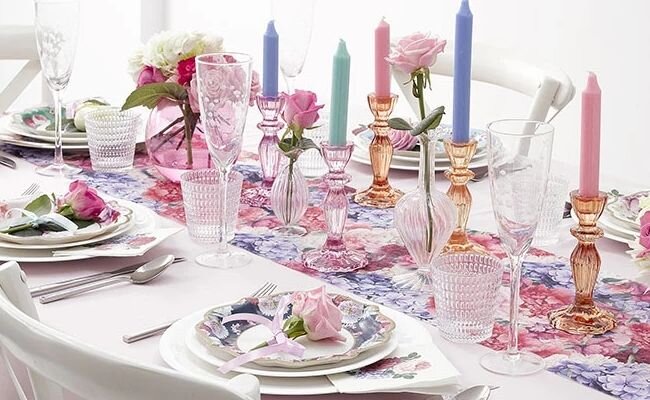The image showcases an elegantly set dining table with a white tablecloth draped over it. At the center, a runner with a pink and light purple floral print adds a touch of color and charm. Surrounding the centerpiece, there are five place settings. Each place setting features a large decorative plate adorned with white flowers and blue accents, creating a harmonious aesthetic. Resting on each plate is a beautiful pink rose tied with a delicate ribbon. Positioned next to the plates, each setting includes a smaller cup and a wine glass.

In the center of the table, amidst the floral runner, candleholders of various colors and designs are arranged. There are two pink candles, three orange glass candlesticks holding two pink and one blue candle, and two pink glass candlesticks supporting one green and one blue candle. Additionally, a small vase containing a bouquet of pink roses adds a final touch of elegance to the table. Towards the top left corner, part of a white chair is visible, completing the picturesque scene.